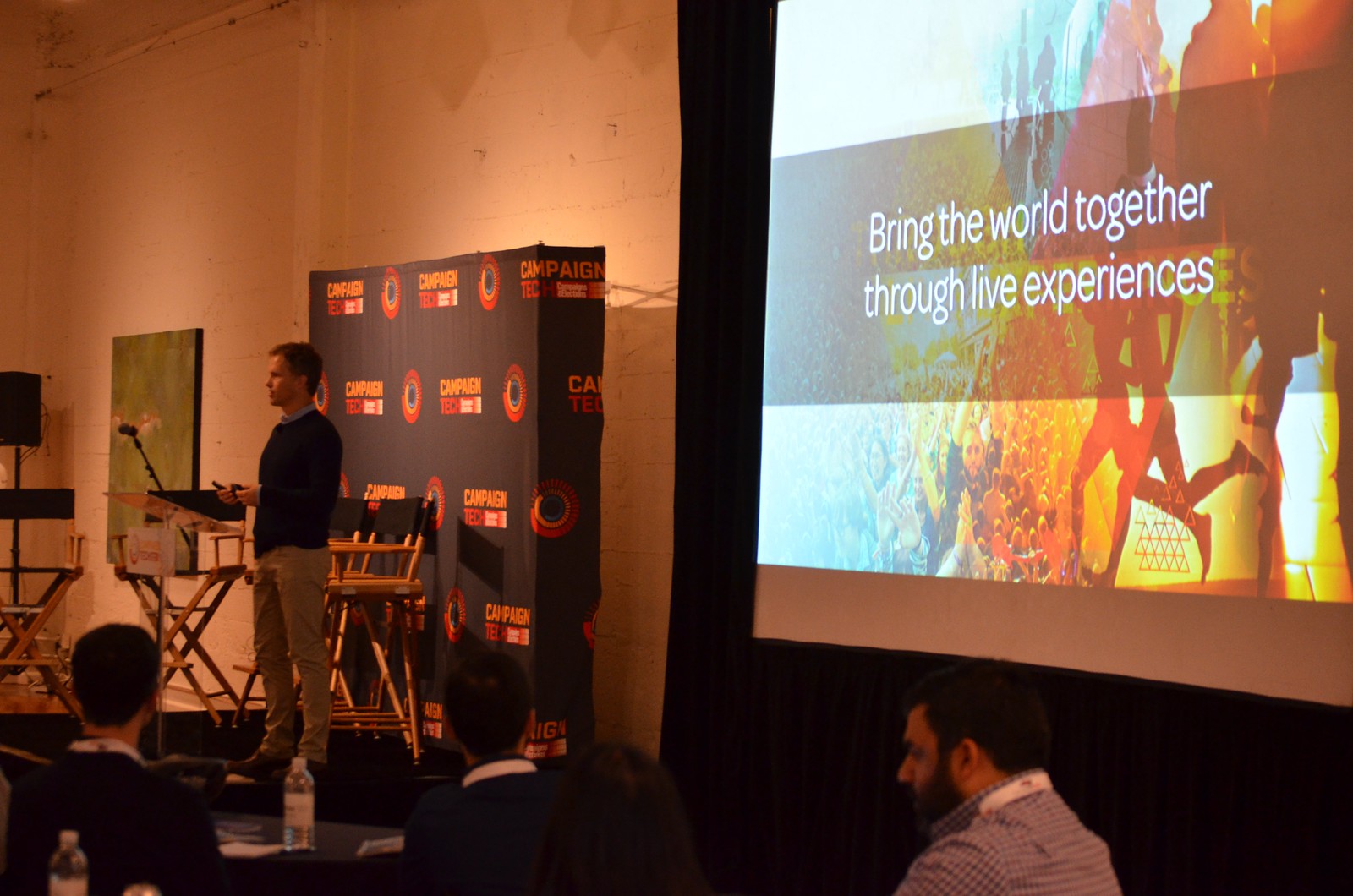The image depicts a somewhat dark photograph of a presentation in progress. The scene is framed horizontally, with the focal point being a small stage area where two director-style chairs are positioned. A white male, wearing a black sweater and possibly khaki pants, stands near the left side of the stage. Behind him is a black banner with a logo that remains unreadable, set against a taller white wall that appears faintly reddish.

To the right of the stage area is a projected image on a white screen that displays a photo of two people running, surrounded by multiple colors—blue, red, yellow, and orange shades—transitioning from light to dark. Across the screen, a horizontal dark band bears the text "Bring the World Together Through Live Experiences" in white.

In the foreground, several audience members can be seen seated at tables. Notably, one table features a bottle and drinks. Seated at this table are three white males: one in a gray suit coat and white collar, another in a black sweater with a white collar and dark hair, and a third individual also in a black sweater. The atmosphere suggests an engaging discussion or presentation, detailed by both the visual elements on stage and the attentive audience below.